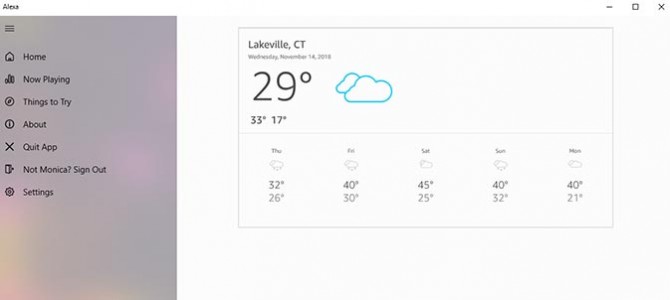This screenshot from the Amazon Alexa platform centers on the taskbar and weather information for Lakeville, Connecticut. The background is primarily a light gray or white, with hints of gray, pink, and yellow along the left taskbar. The left taskbar lists options including Home, Now Playing, Things to Try, About, Quit App, Not Monica, Sign Out, and Settings.

The focal point of the image is a weather widget located in the center, displaying current conditions. The weather is indicated as cloudy, and the temperature reads 29 degrees Fahrenheit. The date provided is Wednesday, November 14th, 2018.